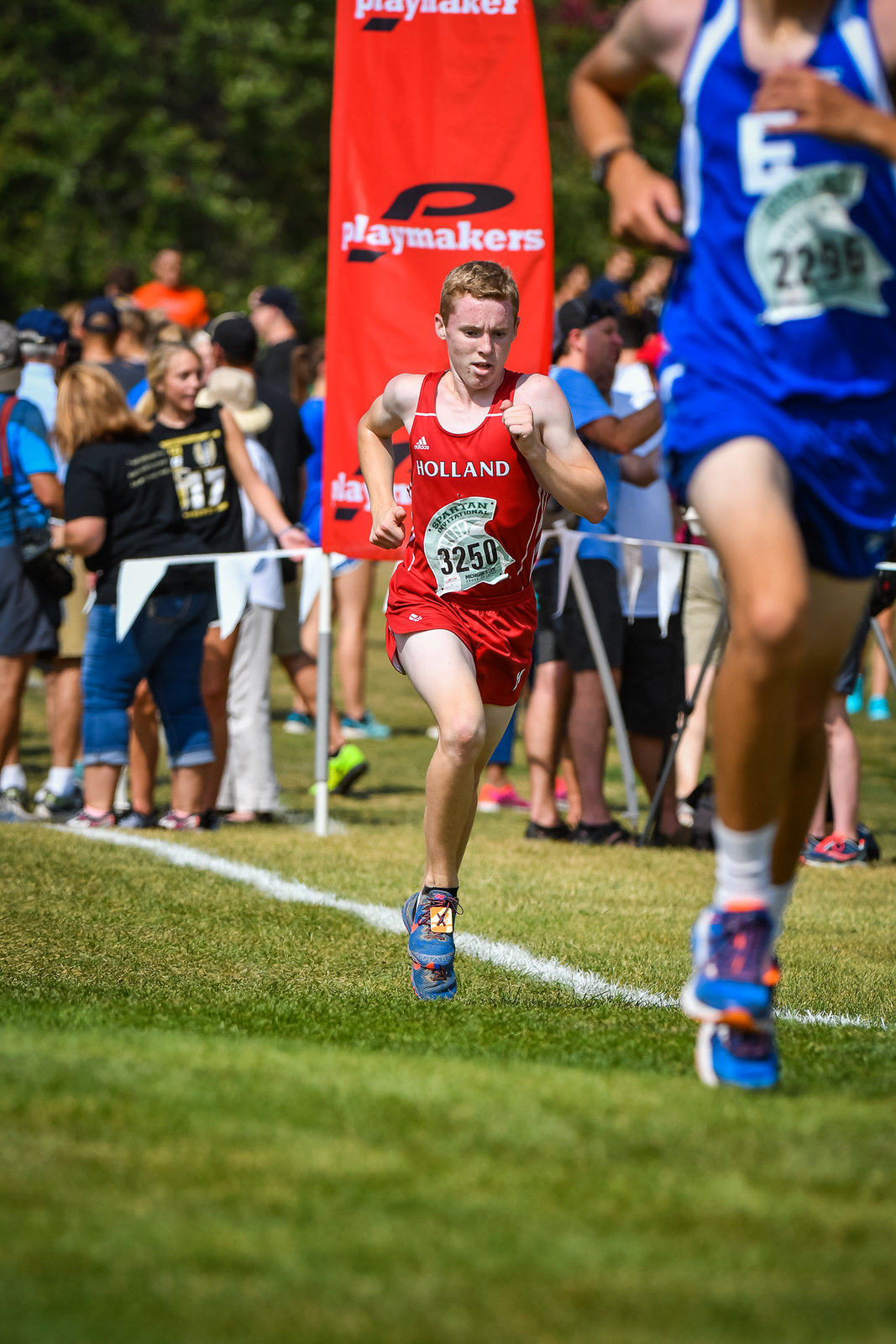The photograph captures an outdoor marathon race, possibly in England, during early evening with minimal shadows. Central to the image is a young white man, likely between 17 to 19 years old, mid-sprint in a red running outfit with "Holland" inscribed on the front, bearing the race number 3250. He appears focused, looking down at the grass beneath his blue running shoes. To his right, another runner in a blue outfit with the race number 2295 is partially visible, just about to exit the frame. The race appears to be held on a grassy course marked by white lines and a flag tape strung across to manage the crowd. In the background, various people are milling around, including a woman in capri jeans on the far left. A red banner with the word "Playmakers" prominently displayed is visible, along with a backdrop of trees.